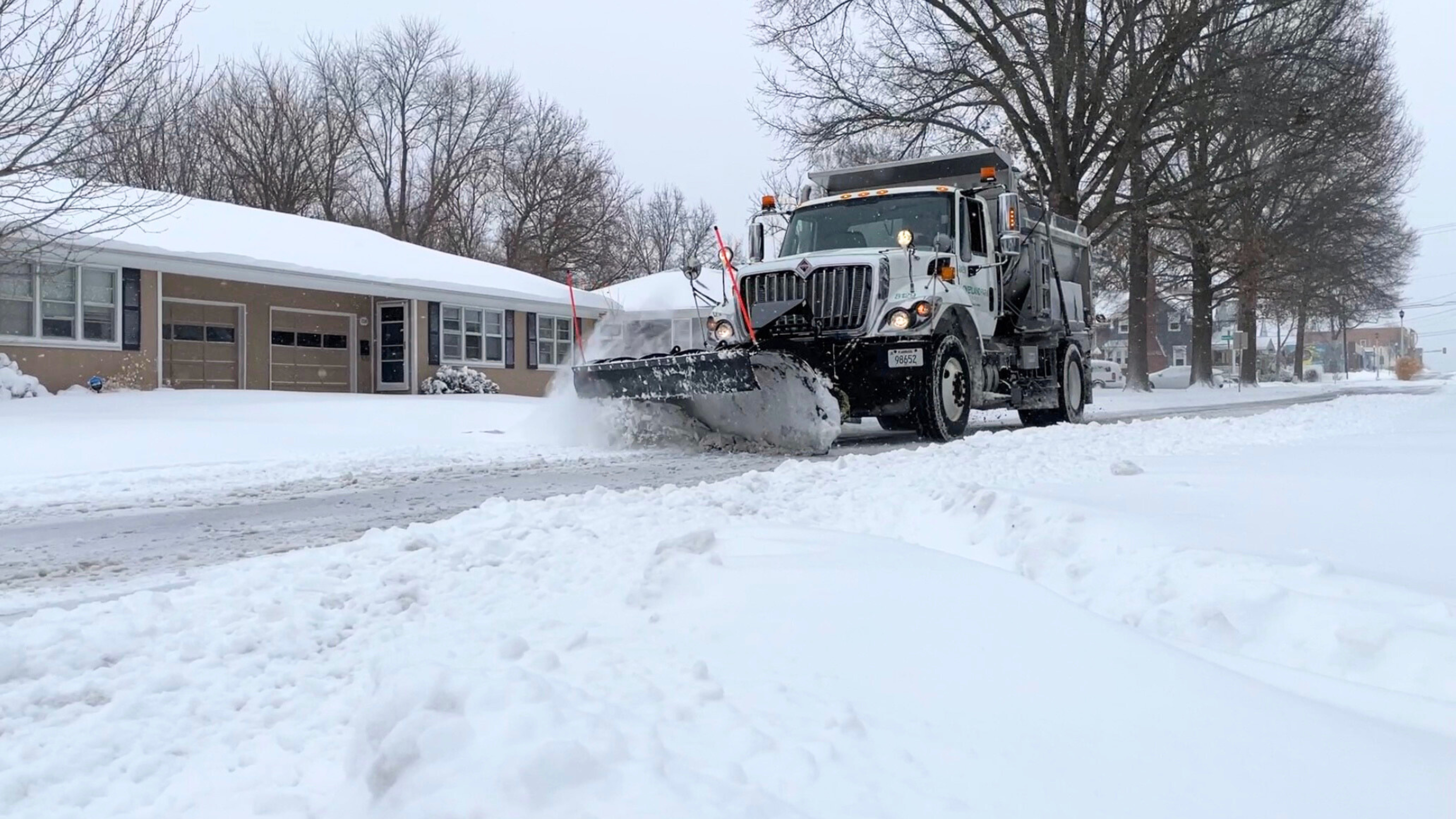In this photograph, we see a snowy city street within a suburban area on a gray, overcast day. The foreground is dominated by a very large, white dump truck equipped with a plow attached to its front. The truck, which features black detailing on its underside and a series of orange safety lights adorning its top, is captured from a low, diagonal angle. Large red poles on the front of the plow help the driver gauge the plow's direction and angle as he attempts to clear a massive clump of snow from the road. The street and surrounding area are heavily blanketed in snow, with snow also covering the roof of a tan, two-car garage home on the left. The house has white-trimmed windows with dark blue sills and sits before a backdrop of leafless, brown trees. The photograph beautifully captures the serene yet challenging winter scene, emphasizing the sheer scale of the snow-clearing operation.